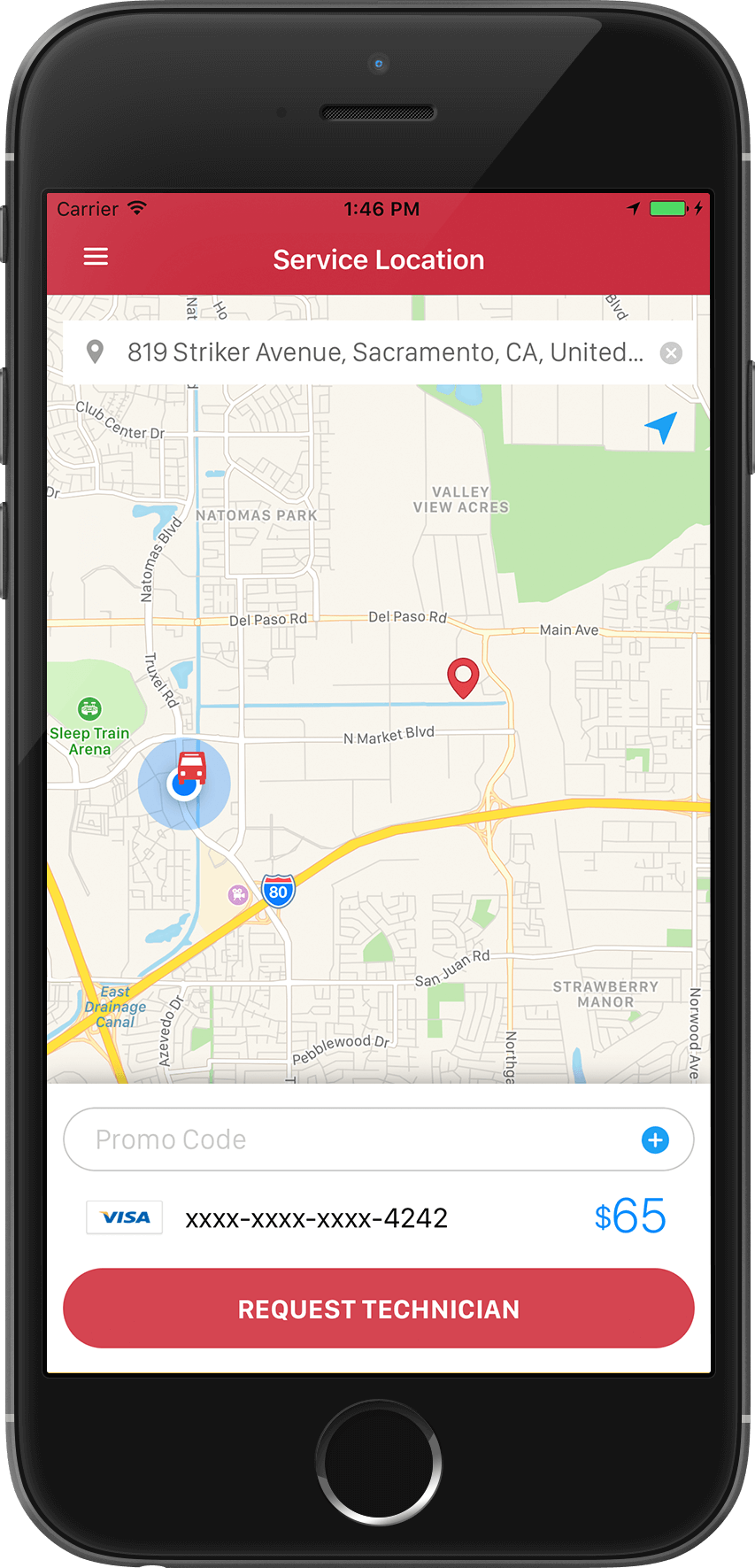The image depicts a cellphone screen displaying a website interface. The phone, noticeably still plugged into a charger, shows it is connected to Wi-Fi, with a battery indicator at full capacity and the time being 1:46 PM. The carrier information is simply stated as "Carrier."

The website on the screen features a map focused on the address 819 Stryker Avenue in Sacramento, California. Below the map, a Visa credit card is listed with the last four digits being 4242, and the service cost is prominently displayed in blue text as $65.

A section allows the input of a promo code, with an associated button featuring a white plus sign inside a blue circle. The website’s color theme includes a red header and footer with white text. At the top, the red header contains white lettering that reads "Service Location" and a menu icon represented by three horizontal white lines for additional options. At the bottom, the red footer has a white text button labeled "Request Technician," situated within a red rectangle.